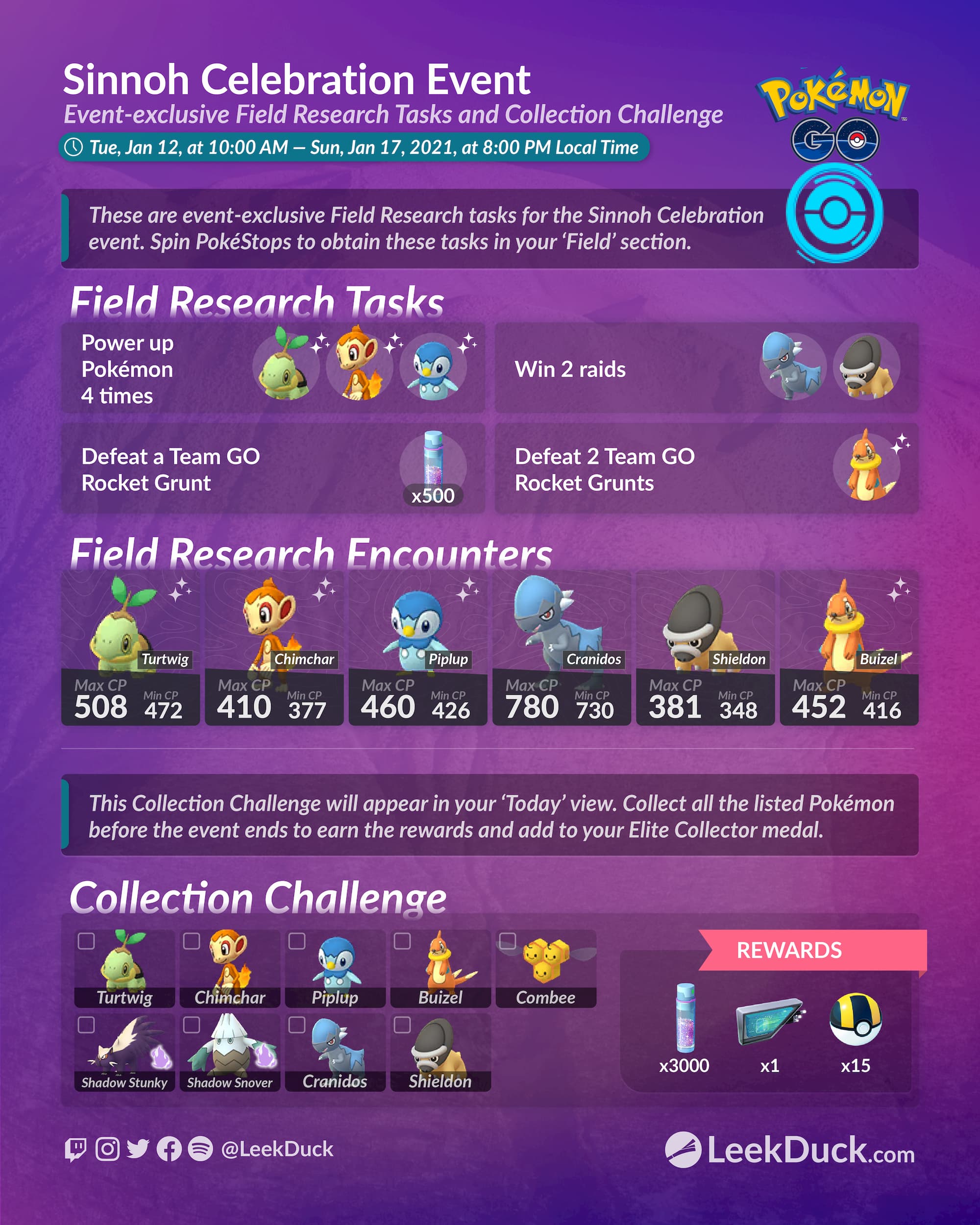**Web Page for Pokémon Franchise: Sinnoh Celebration Event**

The web page features a predominantly purple background, which alternates between shades of purple and lavender. At the center of the page, the header reads "Sinnoh Celebration Event," followed by descriptions about "Event Exclusive Field Research Tasks and Collection Challenge." To the right of the header, the iconic Pokémon logo is prominently displayed, alongside the "Pokémon GO" logo.

Further down the page, contained within a green box, is a clock icon next to the event details: "Tuesday, January 12 at 10 AM through Sunday, January 17, 2021, at 8 PM local time." Below this section, another box elaborates on the event-exclusive field research tasks, which participants can obtain by spinning PokéStops. The text reads: "Spin PokéStops to obtain these tasks in your 'Field' section."

The "Field Research Tasks" section displays four boxes, each containing images of Pokémon and specific tasks:

1. **Box One:** "Power up Pokémon four times."
2. **Box Two:** "Win two raids."
3. **Box Three:** "Defeat a Team GO Rocket grunt."
4. **Box Four:** "Defeat two Team GO Rocket grunts."

Beneath this is the "Field Research Encounters" section, listing various Pokémon characters with their Max CP values. The Pokémon listed include Turtwig, Chimchar, Piplup, Cranidos, Shieldon, and Buizel.

A banner below these sections informs players that the "Collection Challenge" will appear in their "Today" view in the app. Players are tasked with collecting all listed Pokémon before the event ends to earn rewards and contribute to their elite collector medal. The section reiterates that players can check off collected Pokémon from the list.

At the bottom of the page, a series of icons link to various social media and music platforms: a chat icon, Instagram logo, Twitter logo, Facebook logo, and potentially Spotify. The footer text references LeekDuck's website with: "LeekDuck.com – pages from LeekDuck."

Overall, the page serves as a comprehensive guide for participants in the Sinnoh Celebration Event, providing clear details on tasks, encounters, and the collection challenge.